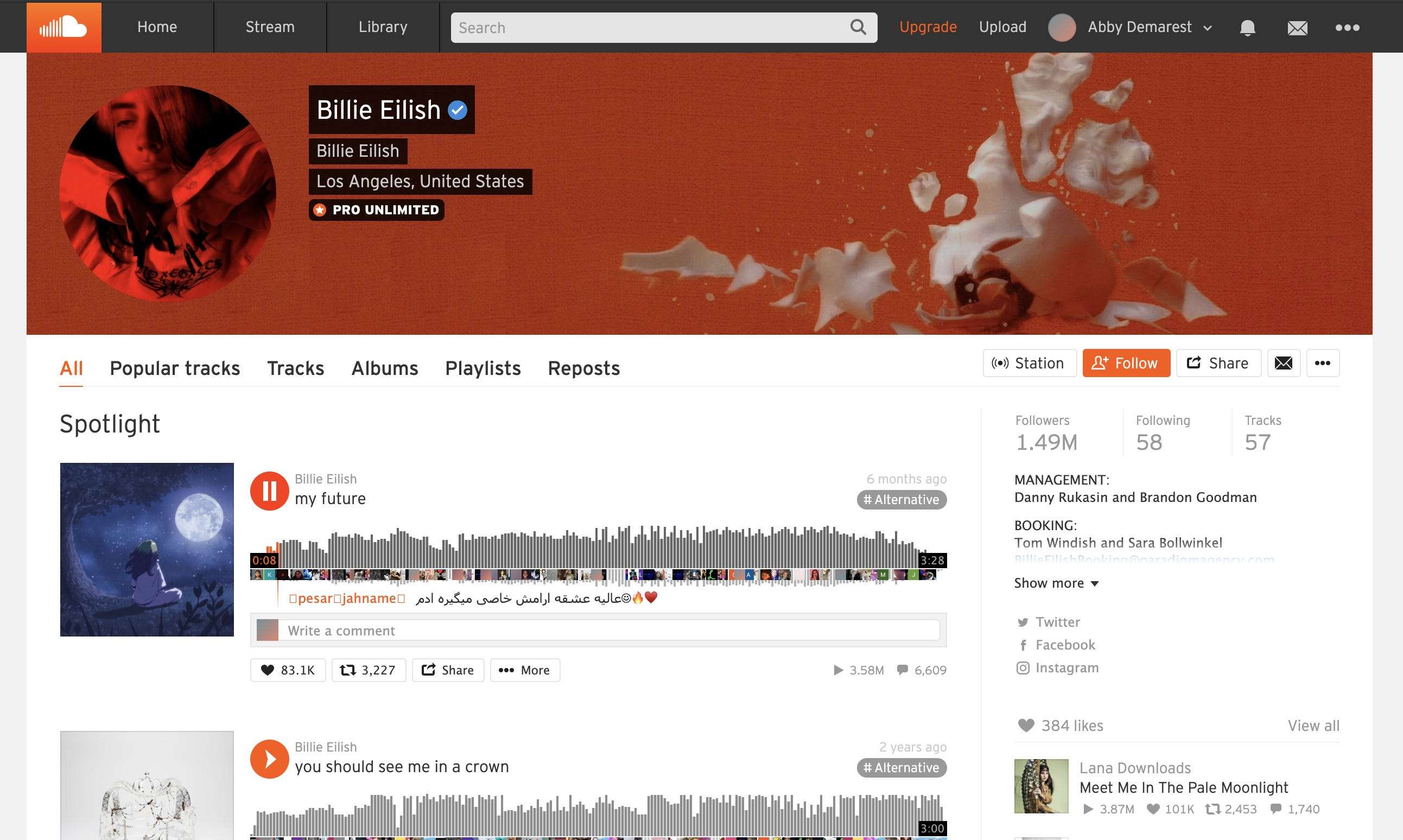In the provided screenshot, we observe a black header at the top featuring the SoundCloud logo on the left. To the right of the logo, the navigation options listed are: Home, Stream, Library, a search bar, Upgrade, Upload, and the user account named "Abby Demarest." 

Below the header, set against a red background, there is an image of Billie Eilish's face. To the right of this image, it reads: "Billie Eilish, Los Angeles, United States, Pro Unlimited." 

Further down, navigational tabs are displayed horizontally from left to right: "All," "Popular tracks," "Tracks," "Albums," "Playlists," and "Reposts." 

Prominently in the spotlight section is Billie Eilish's song "my future." Below this, another song, "you should see me in a crown," is mentioned.

In the upper right corner of the white background, additional details are presented: "1.49 million followers," "Following 58," "Tracks 57." Under management, the names "Danny Rukasin and Brandon Goodman" are listed, while the booking contacts are "Tom Windisch and Sarah Bollwinkle."